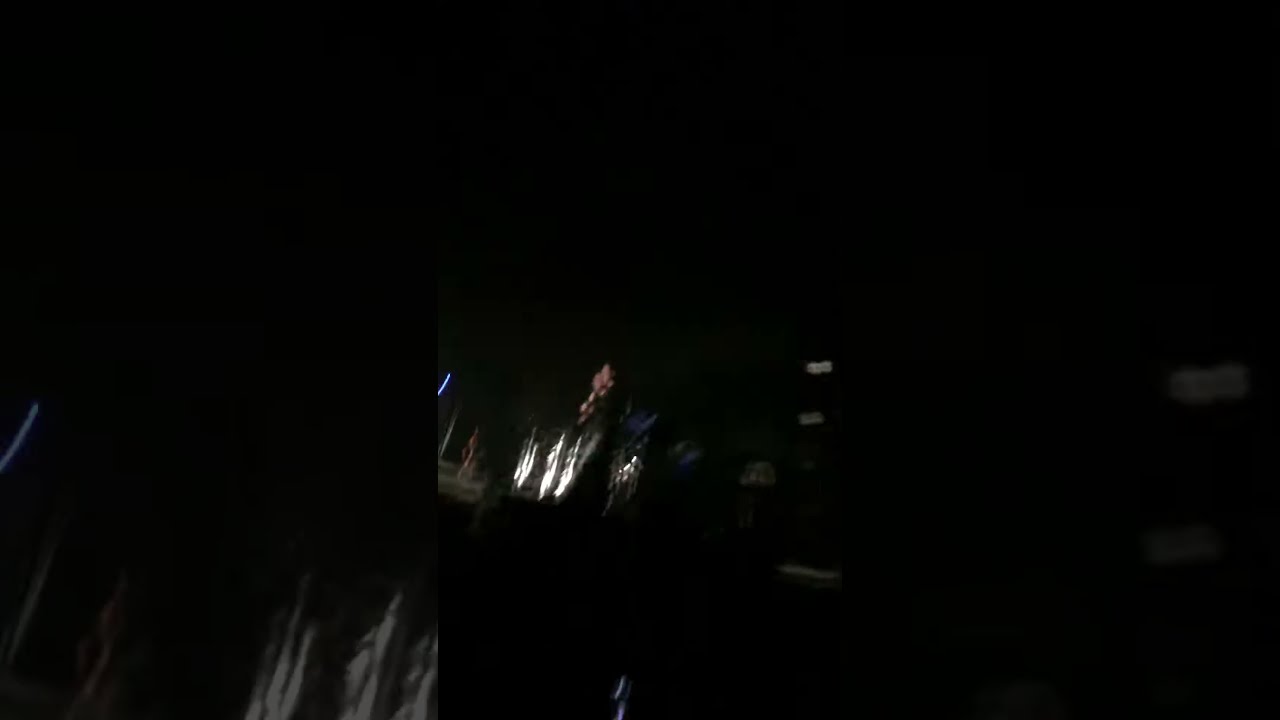The image is predominantly dark, with approximately 95% of it shrouded in blackness. In the center, there's a faint, diffuse light that appears as a smear, suggesting it's an outdoor area with possibly some lights. The left side features smeared gray areas, with one spot showing a bluish tint. Towards the bottom, there are three indistinct, rock-like or tree-like gray smears. On the right side, a couple of barely visible white rectangles can be seen. The middle of the image has various bright streaks and lines, with some white, gray, and bluish hues. There's also a blurry dashed line in the center that appears to have a pinkish hue. Despite these details, the image remains largely indiscernible and very difficult to interpret.